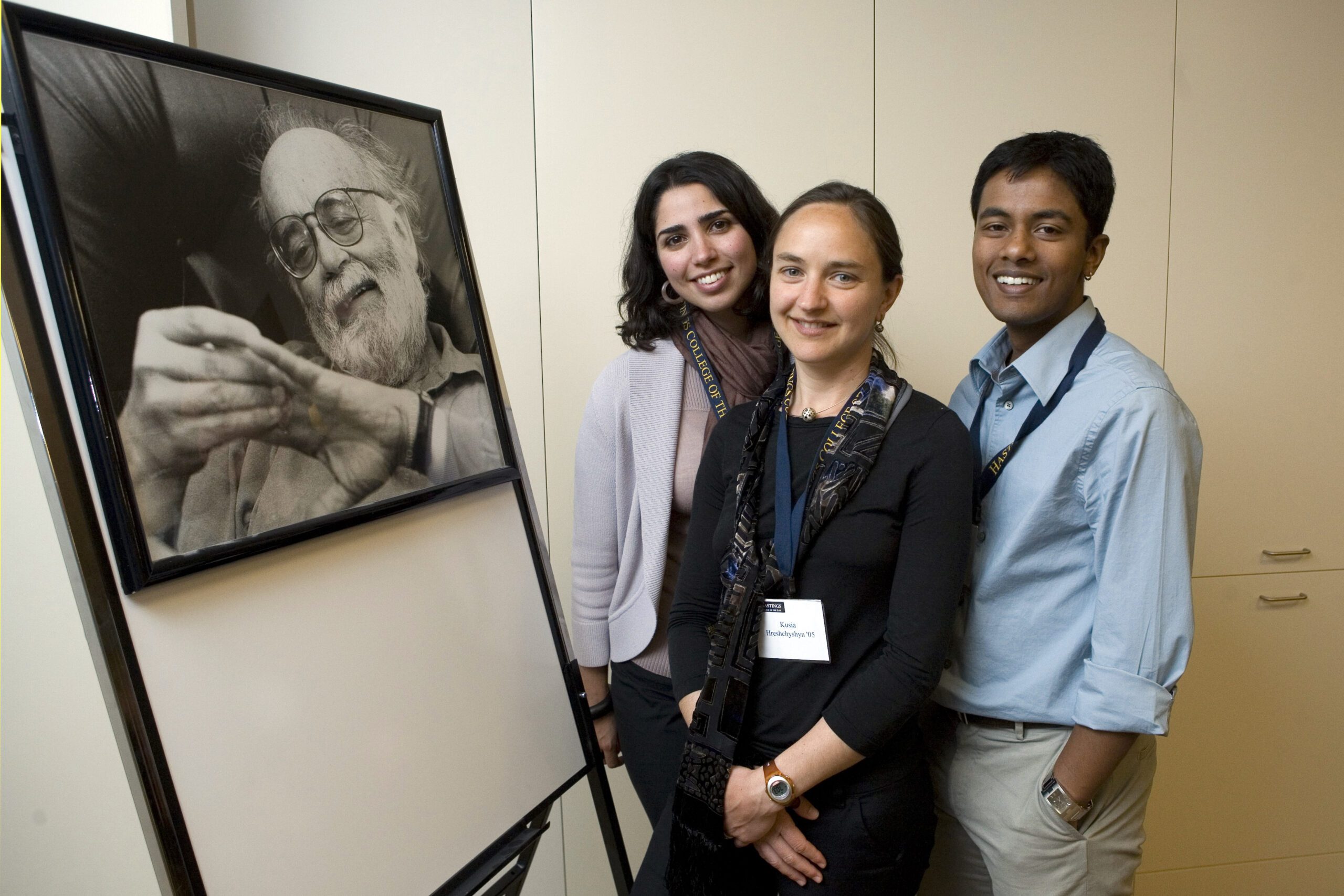In the photograph, three individuals are standing together and smiling at the camera. Behind them are tall white cupboards with silver handles. An easel to their left displays a black-and-white photograph of an elderly gentleman with round-rimmed glasses and a white beard; he is captured fiddling with his hands, giving the image a sense of contemplation. The easel is plain white under the photo.

The central figure is a white female dressed entirely in black with long sleeves that end just above her wrists. She is clasping her hands over her midsection. She wears a watch with a round white face and a brown strap, a navy blue lanyard with a white badge, and a black silk scarf adorned with gold detailing. Her hair is tied back neatly.

Behind her to the left is another woman with dark hair and a bright smile. She wears a white open-knit jumper, black trousers, and a hoop earring, and she has some jewelry on her right wrist. Her lanyard is also navy blue with gold writing. 

To the right of the central female stands a man in a light blue shirt with slightly turned-up cuffs, beige trousers, and a golden rectangular watch on his left wrist. His left hand is in his pocket, and he too wears a navy blue lanyard with gold writing. He smiles warmly at the camera, matching the upbeat and positive energy of his companions.

The group exudes a sense of unity and happiness, as they all wear lanyards that signify a shared affiliation or event, and their collective smiles suggest a moment of camaraderie and celebration.